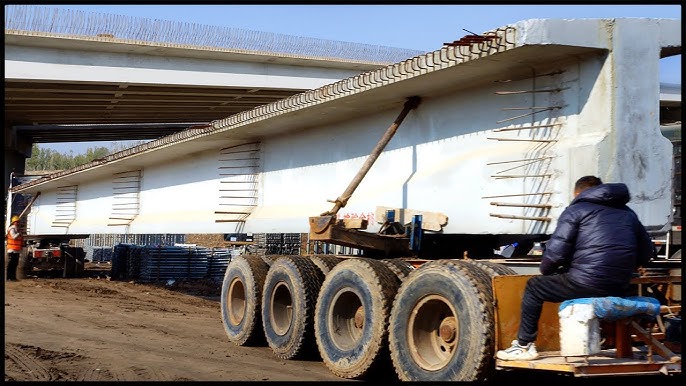This is a detailed photograph capturing the transportation of a large concrete I-beam underneath a bridge on a clear, sunny, cloudless day. The I-beam, which is part of what appears to be an ongoing bridge construction project, is mounted on an extensive trailer featuring large semi-truck-like wheels, with four wheels visible on this side. Positioned at the back end of the trailer is a man in a navy blue winter coat with a hood, dark pants, and white sneakers. He is driving the rear end of the trailer, guiding the concrete beam towards its destination. Another man, wearing a yellow construction helmet, an orange safety vest, and black pants, seems to be directing the operation from the other end of the beam. The backdrop includes a bridge running almost perpendicular to the ground, enhancing the industrial setting of the scene. The ground beneath them is muddy, and there's a distinct lack of clouds in the bright, sunny sky, indicating a clear winter day.